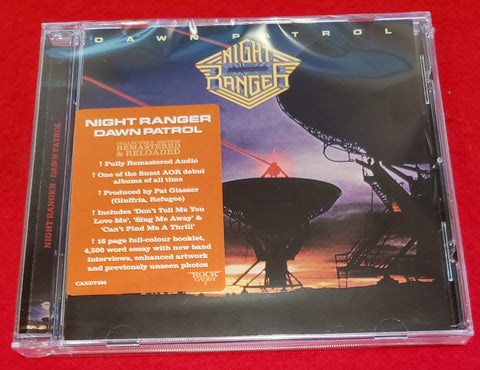This image showcases a retro music CD case for Night Ranger's debut album, "Dawn Patrol." The CD cover art features a dramatic scene with two large satellite dishes, one of which emits a vivid red laser beam into the dusk sky. The backdrop transitions from a sunset-orange horizon to darker clouds above, creating a striking contrast. Prominently placed on the cover is a yellow shield-like emblem with the band name "Night Ranger" in bold yellow text. An orange sticker on the cover provides additional information, including, "Night Ranger Dawn Patrol, fully remastered audio, one of the best AOR debut albums of all time," and it lists notable tracks like "Don't Tell Me You Love Me," "Bring Me Away," and "Can't Find Me a Thrill." The left side of the CD case also features a label with similar promotional text. This special edition includes extras like an 11-page full-color booklet, a comprehensive 4500-word essay with new band interviews, enhanced artwork, and previously unseen photos, making it a treasure for fans and collectors alike.